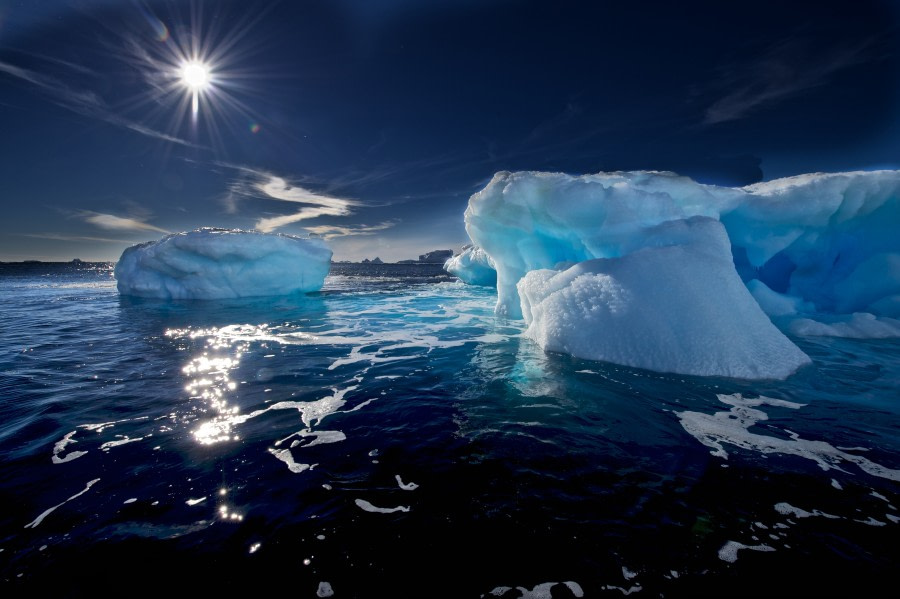In this captivating night-time Arctic seascape, a deep, dark blue ocean stretches out under a similarly dark blue sky, with the view dimly illuminated by a large moon in the upper-left corner. The tranquil sea is dotted with floating icebergs and patches of white foam. The largest iceberg, positioned near the center-left of the image, is a vast, gleaming white formation tinged with light blue hues. Two additional, towering icebergs can be seen on the right, casting reflections on the calm, vivid dark blue water. Wispy white clouds adorn the sky, adding a touch of ethereal beauty. In the distant horizon, partially shrouded by a misty sheen, lies a faint silhouette of trees or a cityscape. The moonlight creates a silvery path across the water, enhancing the serene and otherworldly atmosphere of this Arctic wonderland.